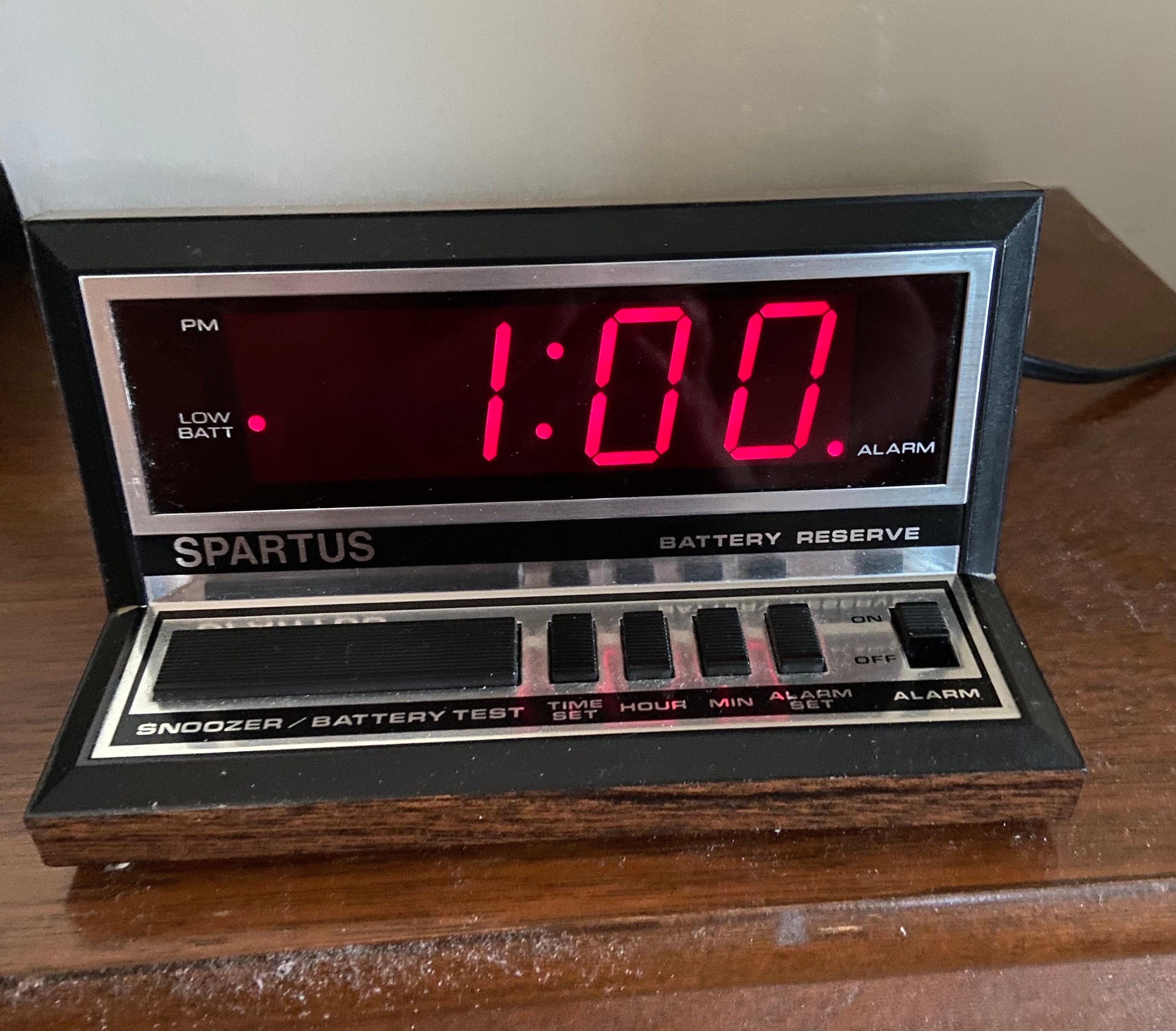This image displays an old digital alarm clock prominently positioned on a medium to dark brown wooden nightstand or dresser, which is noticeably dusty and scuffed. The alarm clock itself features a stark black plastic border with a silver faceplate. The time is shown in bold red digits, reading 1:00 PM, with a lit indicator for low battery on the left side and an alarm set indication on the right. Detailed buttons and labels are present at the bottom, including "snoozer/battery test," "time set," "hour," "minute," "alarm set," and an "on/off" switch for the alarm. The brand name "Spartus" is displayed above these controls. A visible black cord extends from the back of the clock towards the right side, against a backdrop of a white wall with a faux wood border near the bottom edge. The overall appearance suggests that both the clock and the surface it rests on have seen better days.